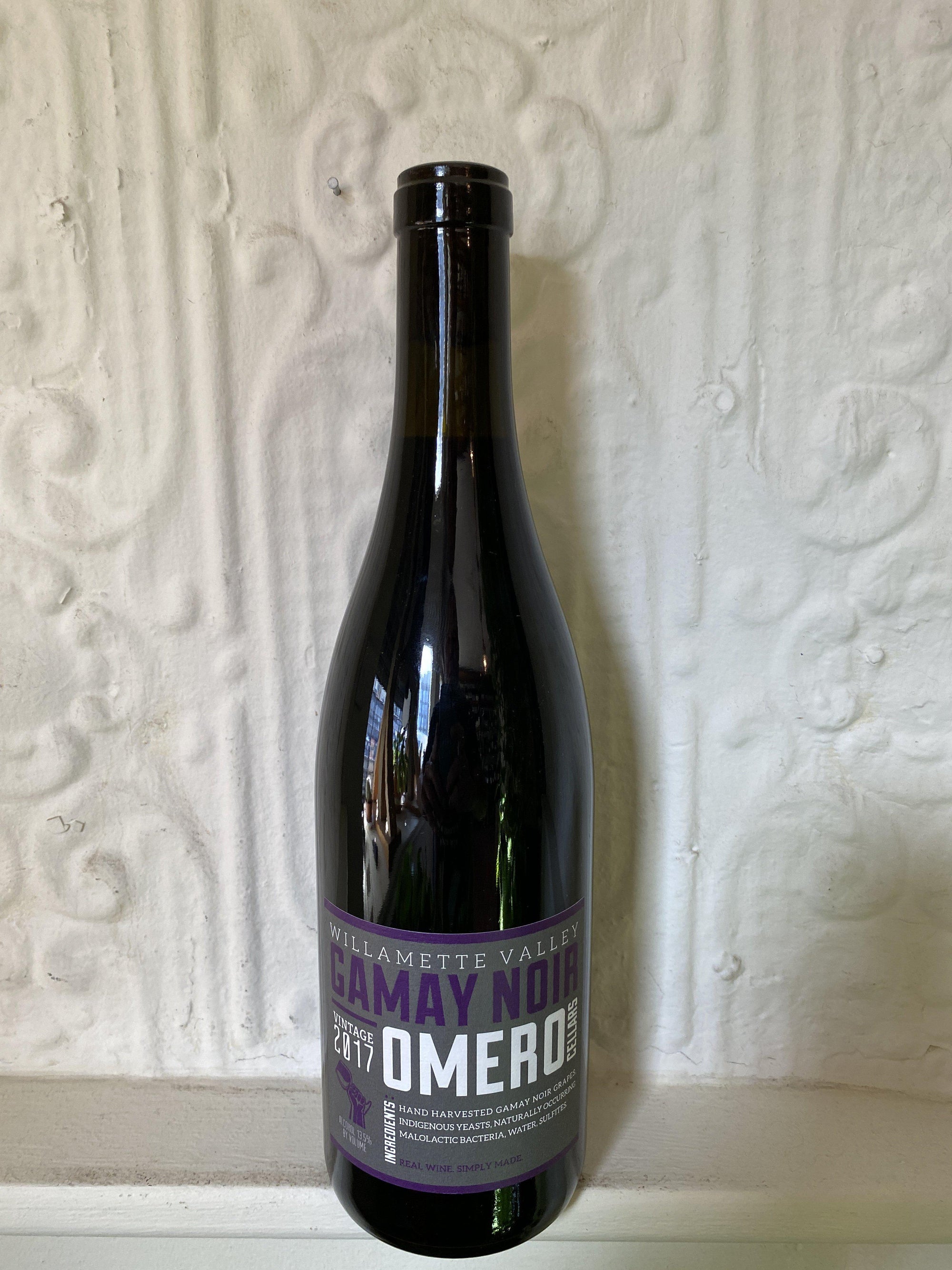This intricate illustration depicts a dark, glass wine bottle positioned on a narrow white wooden ledge, set against a detailed plaster wall adorned with raised moldings. The bottle's body is nearly cylindrical with a long, slender neck. It features a distinctive light purple label with both white and dark purple text, some of which reads "Willamette Valley," "Gamay Noir," "Vintage 2017," and "Omero Casitas." The scene captures a hint of sunlight reflecting off the bottle, suggesting the presence of windows nearby. Notably, the bottle appears to be empty, as it lacks both a cork and a cap.